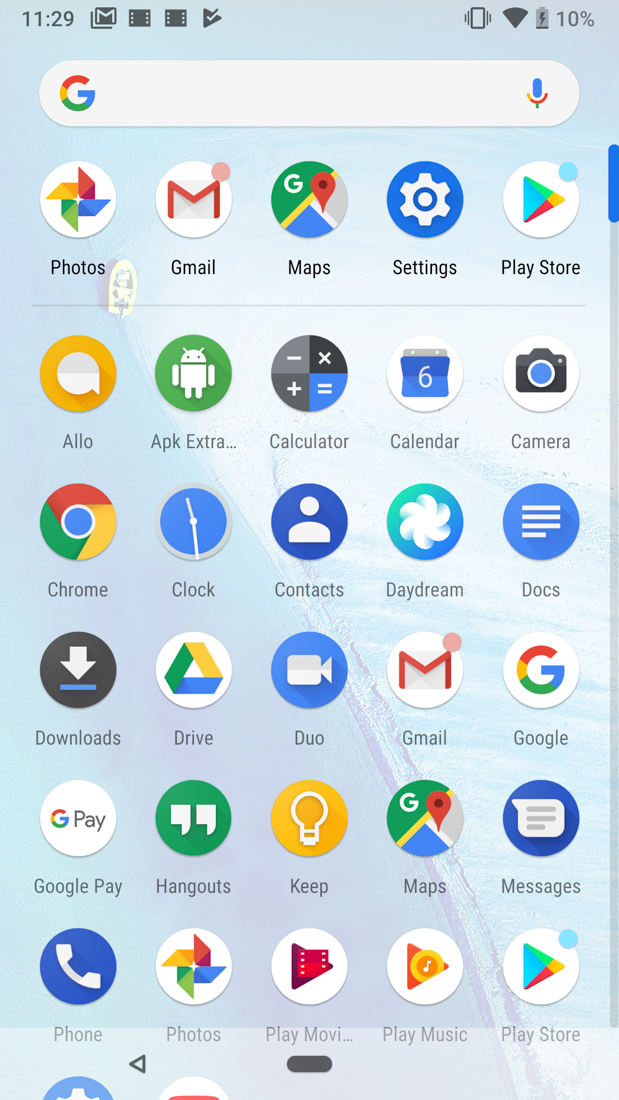Screenshot of a smartphone displaying a vibrant ocean-themed wallpaper with a white boat sailing towards the top left. In the status bar at the top, the time reads 11:29 AM, and there is a Google Mail notification icon. The phone is on vibrate mode, as indicated by the icon on the far right, and it is connected to Wi-Fi with a battery level at a critical 10%. Below the status bar is a Google search bar, followed by a grid of app icons.

Starting from the top left, the visible app icons are: Photos, Gmail, Maps, Settings, Play Store, Allo, APK Extra, Calculator, Calendar, Camera, Chrome, Clock, Contacts, Daydream, Docs, Downloads, Drive, Duo, Gmail, Google, Google Pay, Hangouts, Keep, Maps, Messages, Phone, Photos, Play Movies, Play Music, and Play Store. Additional app icons are located at the bottom, but they are partially cut off, making them difficult to identify.